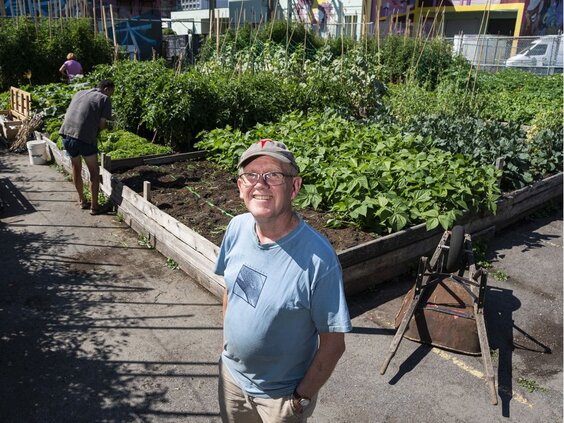This rectangular, color photograph captures an outdoor community garden scene with a clearly visible older gentleman posing and smiling in the center. The man appears to be around 60 years old and stands prominently, pictured from head to mid-hip, wearing a beige (or khaki) baseball cap, wire-rimmed glasses, a light blue t-shirt, and light brown (or khaki) pants. His hands are casually tucked in his pockets, and he looks up toward the camera, beaming with a warm smile. Behind him, the garden is filled with several raised beds framed in light-colored wood. Each bed contains patches of dark soil and green plants, indicating a mix of thriving plants and freshly planted areas. 

To the man's right, an upside-down wheelbarrow lies on the ground, and to his left, the garden extends further, showing more intricate sections on a gray pavement. In the background, two other people are engaged in gardening, bent over different raised beds. One wears a black jacket and shorts and faces away from the camera, while the other, positioned further back, is also tending to the garden with parked vehicles visible in the distance. A short stepladder with a brown bag underneath it can be seen on the bottom right. The overall scene evokes a sense of peaceful engagement with nature, captured in a moment rich with photographic realism.